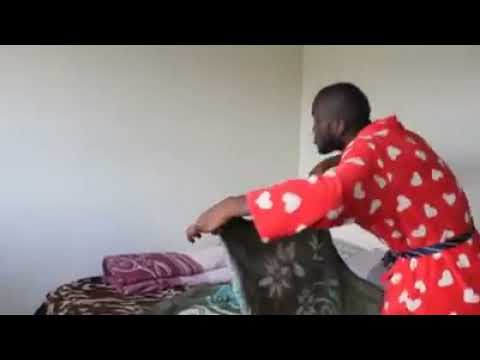In a softly lit room with blank white walls, a dark-skinned man with very short or no hair and a beard is captured mid-action. He is dressed in a striking red bathrobe adorned with white hearts, cinched at the waist by a blue striped belt. The man, positioned sideways, is hunched over a bed, meticulously folding or placing an olive-green rug with white floral patterns. The bed is scattered with other textiles, including a distinctly folded red and white item and a purple piece. The photograph, though somewhat blurry with black bars at its top and bottom, captures the man's focused expression as he works intently with the green rug in his hands. Natural light filters into the space, providing a gentle, ambient illumination that highlights his concentrated demeanor.